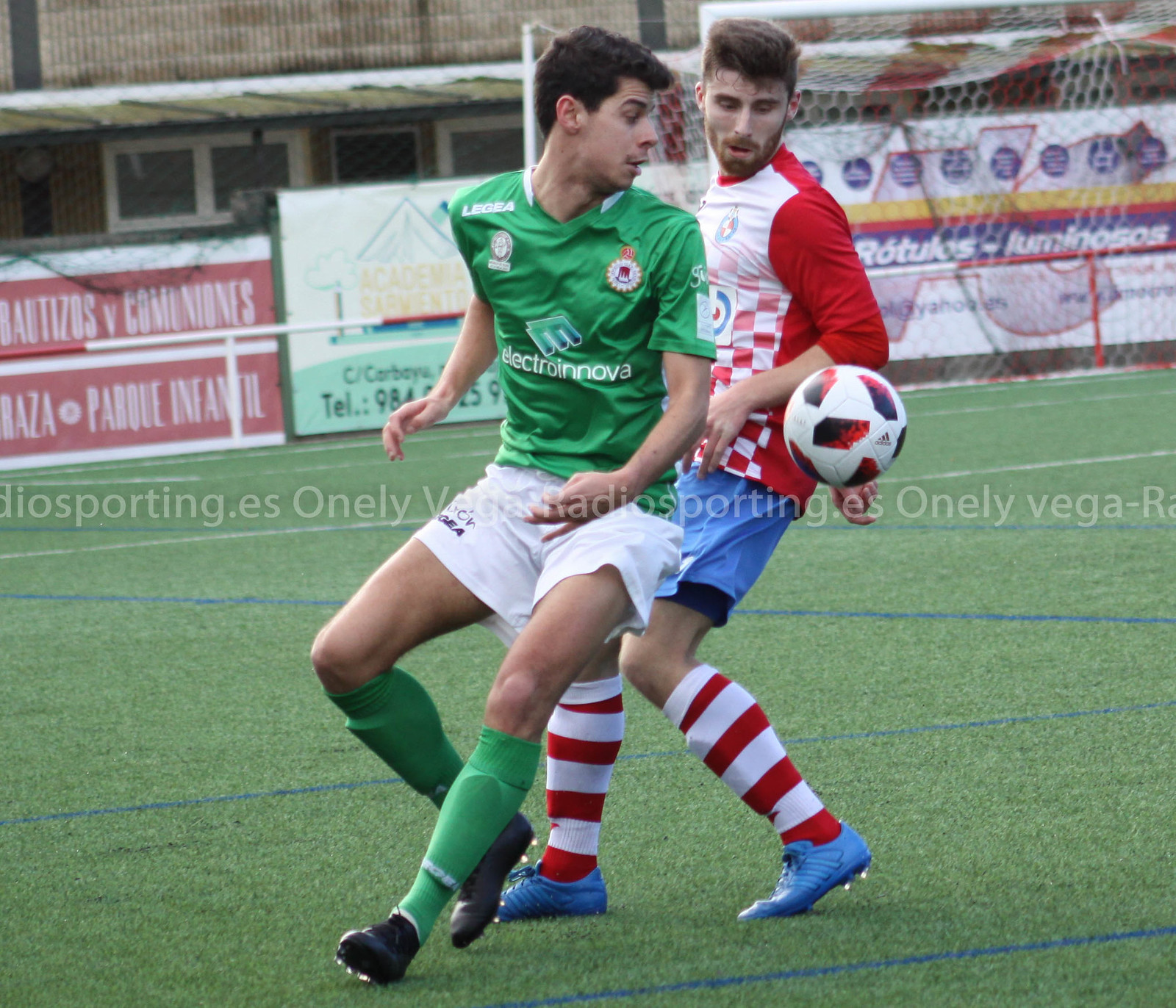In the image, two soccer players are mid-action, seemingly competing for the ball, which is suspended in midair between them. The player in the foreground is glancing back over his shoulder, dressed in a green uniform with green socks pulled over his shin guards, white shorts, and black shoes. Behind him, another player is attired in a red and white checkered jersey with a plain red back, blue shorts, red and white striped socks, and blue cleats, looking to his left. The field they are on has a green surface with blue and white boundary lines. In the background, you can see various banners with red, white, and green text, along with telephone numbers and partially legible words, including "radiosporting.es" and "only Vega." A soccer goal is visible behind the two players, adding context to their dynamic engagement.